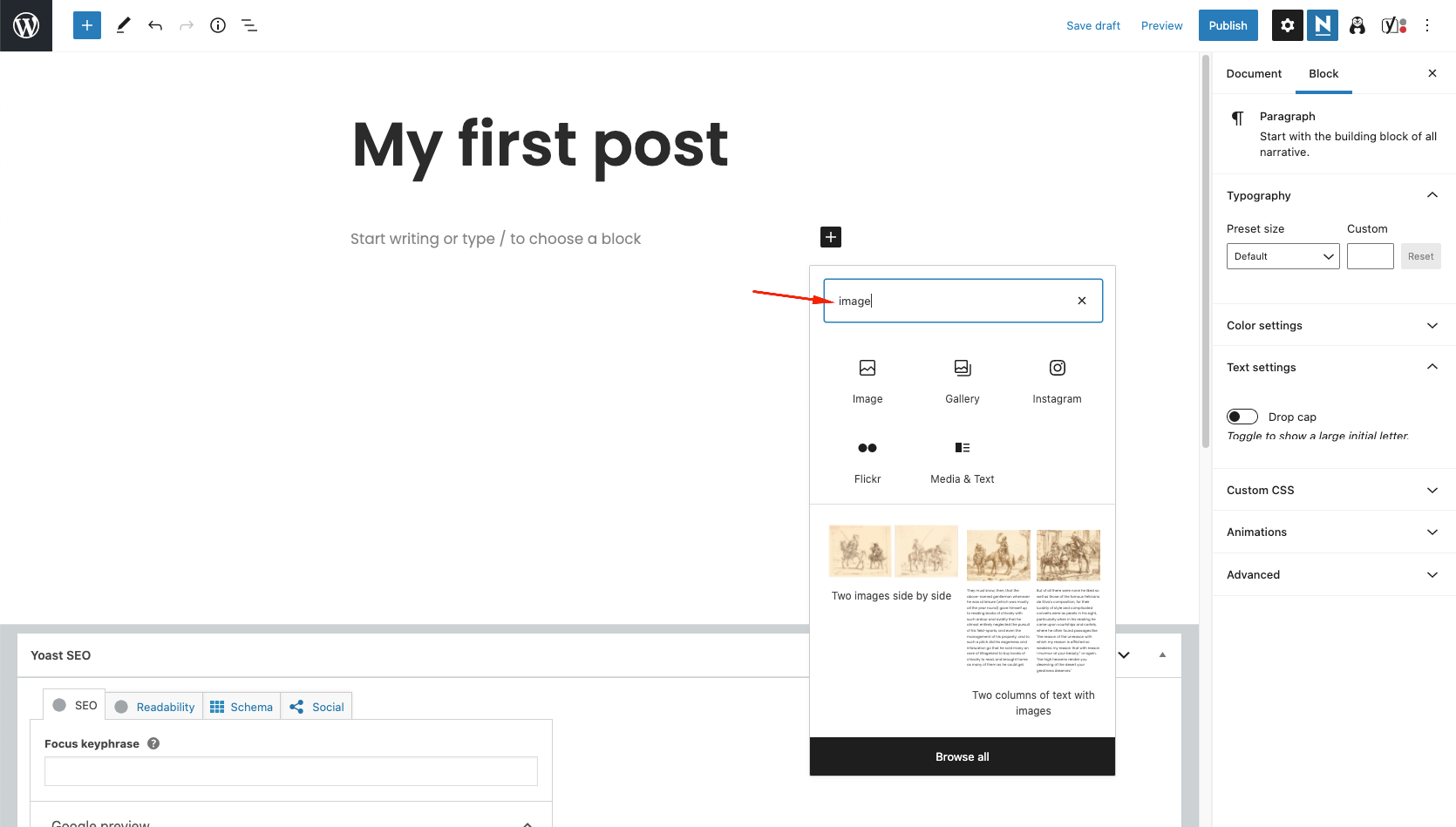A detailed screenshot captures the WordPress dashboard interface, illustrating the steps for creating a first post. Dominating the image, a bright red arrow draws attention to the field labeled "Image," emphasizing the visual element of the post. The dashboard itself is primarily white, providing a clean and uncluttered background. In the far-left corner, the recognizable WordPress logo is prominently featured for brand identification. Gray dialog boxes scattered around guide the user with pertinent information, and a right-hand sidebar offers various command options. At the bottom, a black bar labeled "Browse All" invites further exploration of available features. The overall layout is straightforward, designed to assist users in navigating the complexities of their inaugural WordPress post.